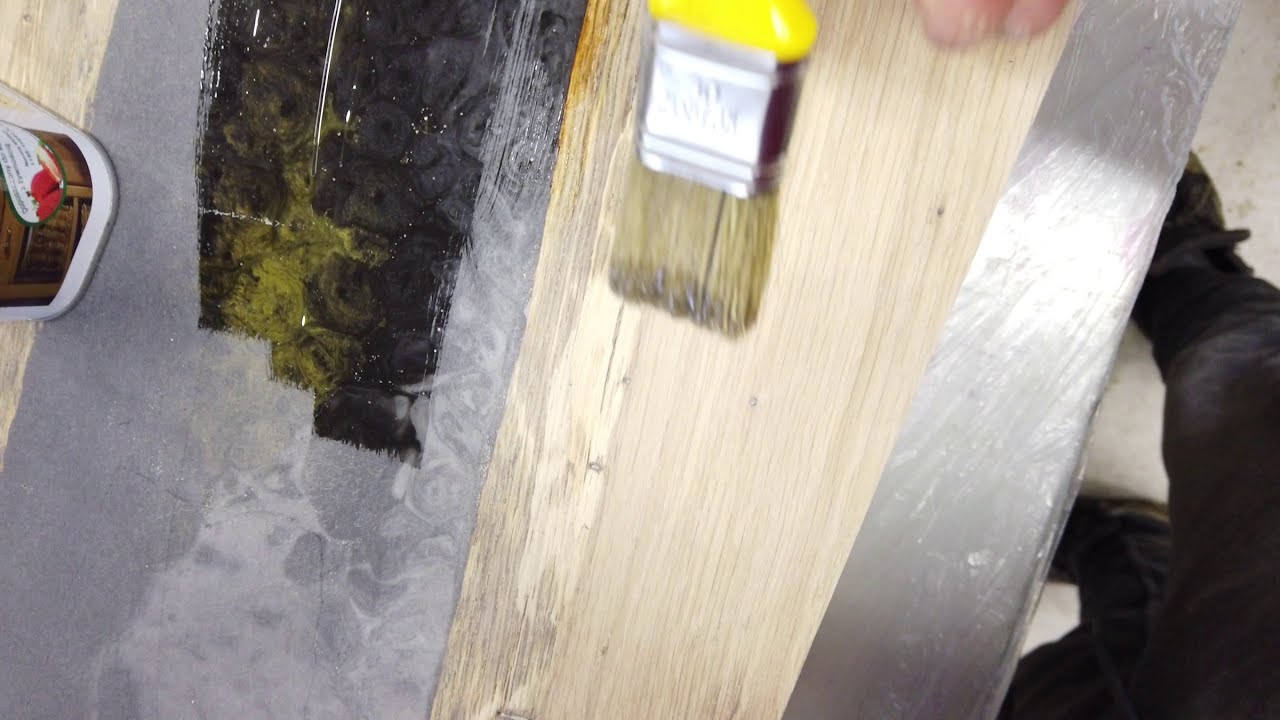The image depicts a detailed, horizontally oriented close-up scene centered around a paintbrush with a yellow handle, a silver bezel, and natural-colored bristles. The paintbrush lies horizontally across a natural piece of wood located in the top center of the image. Dark black paintbrush strokes are visible on a light gray concrete surface to the left of the wood. Toward the right, a metallic strip can be seen. In the lower right corner, a person's legs clad in dark black pants and black shoes stand on a light-colored floor, implying their involvement in the painting process. The upper left corner reveals a glimpse of a white can adorned with a brown and red sticker, which may contain paint or wood care products. The setting is well-lit, highlighting the textures and details of the wooden board and the various elements in the scene.